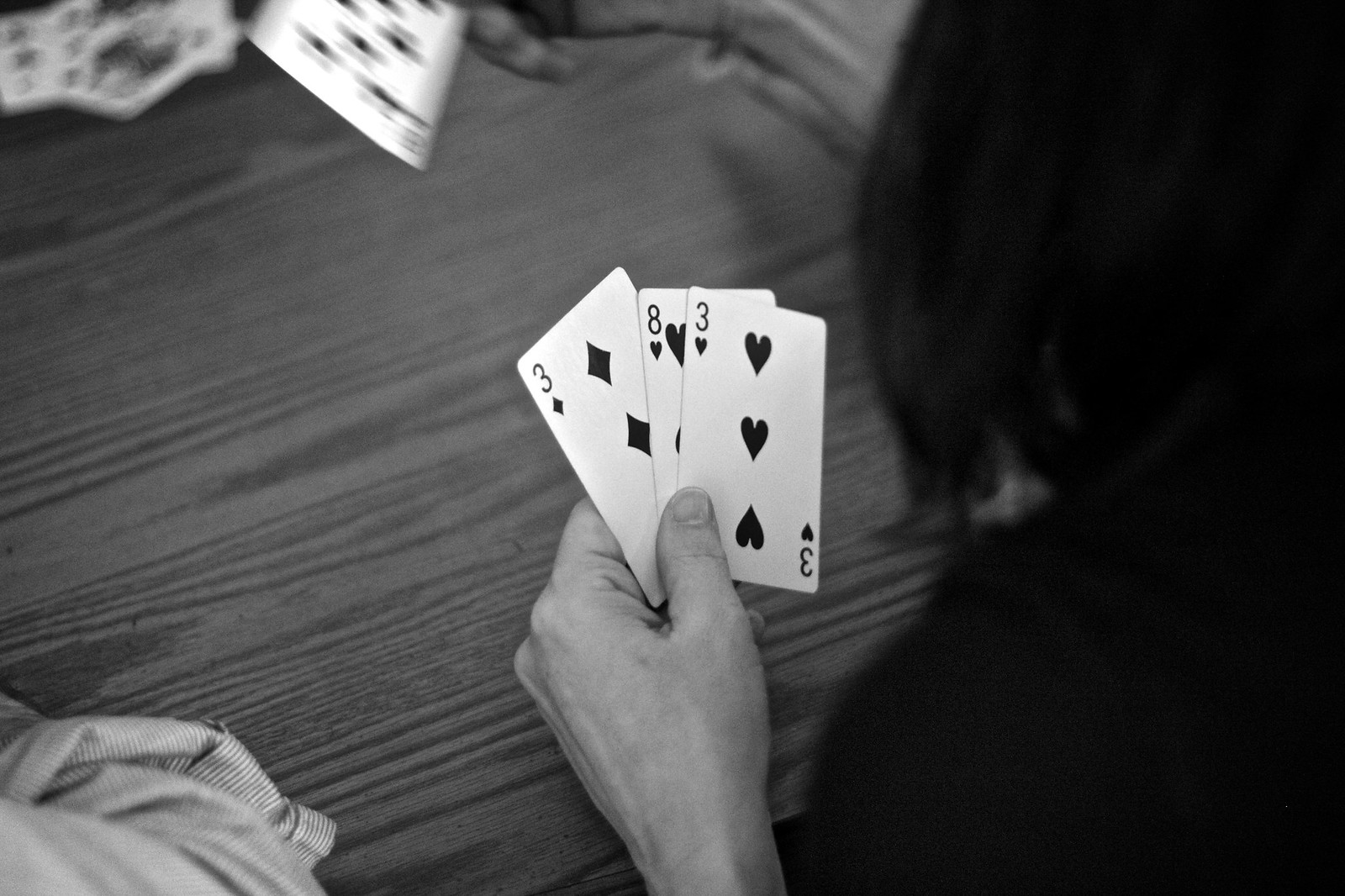In this evocative, black-and-white photograph, the focus is on a person engrossed in a card game. The image is captured from behind and slightly over the person's shoulder, creating an intimate and almost voyeuristic perspective. The individual in the foreground is donning a black hoodie, with their straight, black hair cascading just below their shoulders, effectively obscuring their face from view. Their left hand, poised at the edge of a wood-patterned table, holds three playing cards in a staggered, fan-shaped arrangement: a three of diamonds, an eight of hearts, and a three of hearts.

Just visible at the top edge of the photograph is the person's right hand, partially out of frame and blurry, seemingly in mid-action, holding an eight of clubs. The composition centers sharply on the left hand and its three cards, while the surrounding elements—such as a stack of face-up cards in the upper left corner and the indistinct gray-and-white striped fabric of someone's rolled-up sleeve in the lower left—remain softly out of focus. The blurred background contributes to the intimate and mysterious atmosphere of the scene. The photograph, horizontally aligned and rectangular in shape, captures a fleeting, silent moment in the timeless tradition of playing cards.